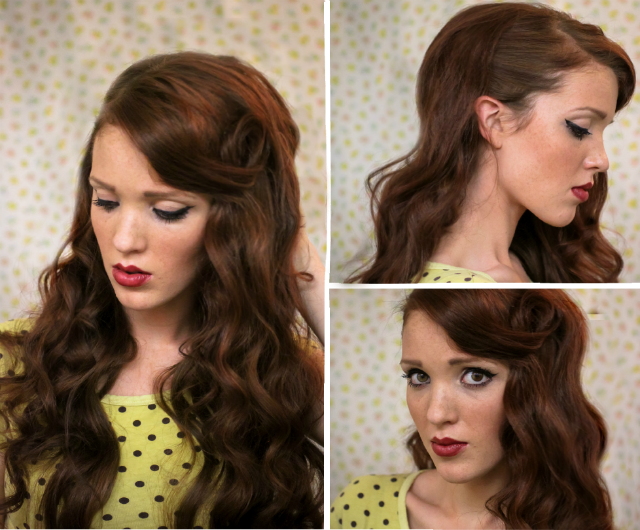The image is composed of three distinct photographs of the same woman, arranged on a single magazine page. The left side features a larger, elongated image, while the right side contains two smaller photographs stacked vertically. The woman has long, dark auburn hair, blending curly and straight textures, cascading down and adorned with reddish highlights. She wears a bright yellow dress with small black polka dots and has a noticeable makeup application, including dark red lipstick, eyeliner, mascara, and a hint of blush, enhancing her delicate freckles.

In the larger left photograph, she is posed with her hand behind her head, looking downwards towards the bottom left, giving an introspective expression. The background behind her is dynamic, filled with scattered multi-colored dots in yellow, red, and blue. On the right side, the top photograph captures a side profile of her face, where she is looking downwards with her eyes mostly closed, and her hair is pulled back to reveal her right ear. The bottom photograph on the right presents her facing the camera directly, her dark eyes engaging the viewer with a sullen yet captivating look.